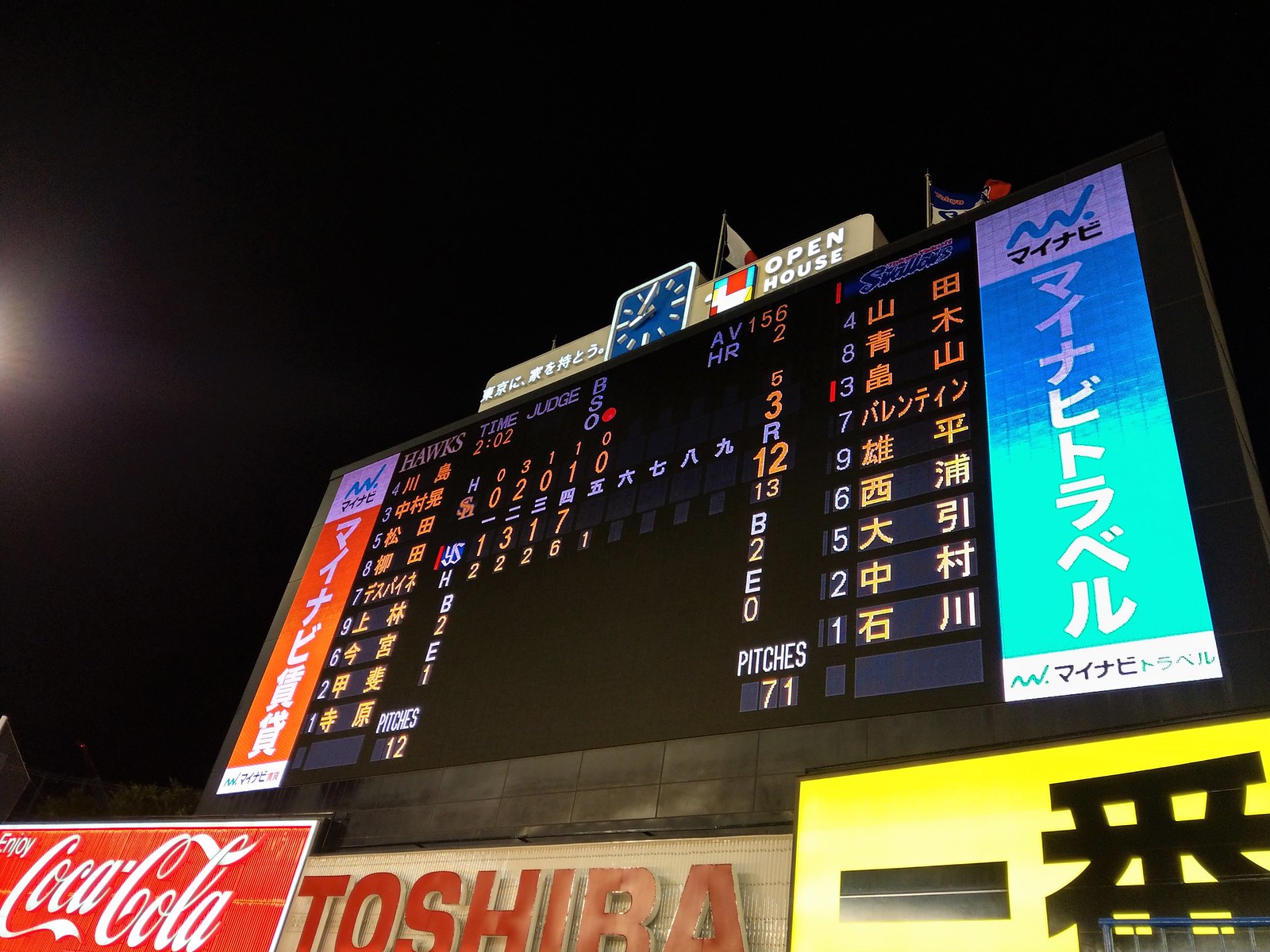This is a horizontal rectangular photograph of an electronic scoreboard, taken at night, evident from the black background. The scoreboard, situated in a Japanese baseball stadium, is adorned with Japanese characters and displays the game’s progress. Prominently in the center, the scoreboard's blue clock reads 9:05, indicating the game is in progress at night. It also provides details such as the number of pitches, which are visible at the lower right and left corners.

The scoreboard reflects the game between the Hawks and another team starting with an "S". The current score shows five runs for one team and three runs for the other, with the game in the seventh inning. The surrounding area is filled with various advertisements: to the bottom left is a Coca-Cola sign, next to it in the middle is a Toshiba advertisement, and to the right is an ad in black characters on a yellow background. Additional advertisements flank the scoreboard on either side, although they are not legible. Above the scoreboard, you can see a Japanese flag waving, adding to the ambiance of the scene captured from a lower right vantage point.